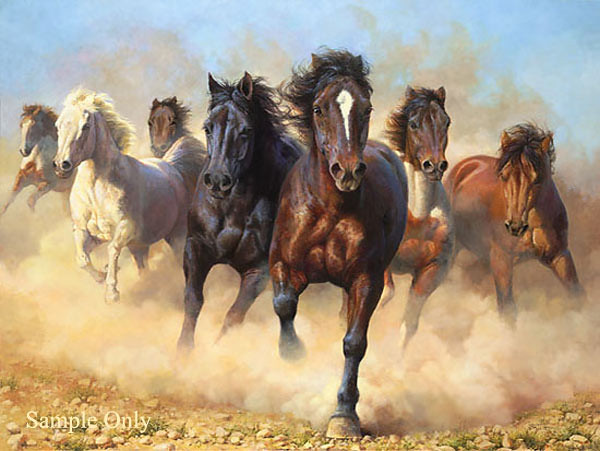The image depicts a detailed painting of seven galloping horses, moving energetically towards the viewer, creating an almost surreal scene with dust clouds swirling around them as they traverse rocky terrain. The sky above them is a clear blue, providing a striking contrast to the earthy tones of the ground. Starting from the left, the first horse is a striking pinto with white and brown patches. Next is an all-white horse, slightly behind it. Following is a brown horse, of which only the face can be clearly seen. To its side is a dark brown, nearly black horse. The central figure is a robust brown horse with grey legs and a distinctive white marking on its face. Next, another pinto, showcasing a white and brown mix. Finally, on the far right, stands a deeply rusty brown horse. The painting's composition is further marked by the text "sample only" in white lettering at the bottom left corner.